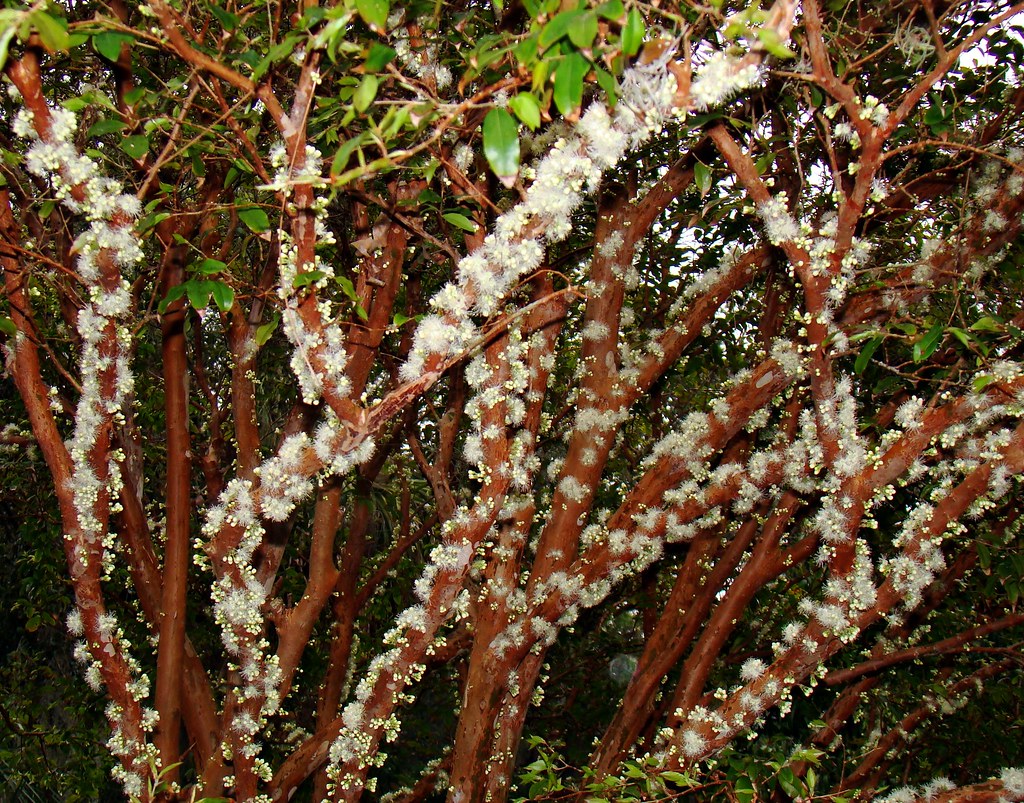This image captures a detailed close-up of a shrub-like plant situated in a dense, leafy forest setting. The central plant features several medium to thick brown branches that climb vertically, occupying the entire height of the image. These branches are extensively covered in a white, cottony substance that resembles dandelion fluff or cotton balls, lending a mossy appearance. Interspersed among the white fluff, near the ends of the branches, are small green leaves and budding flowers, suggesting that these white formations could be related to seed dispersion. The background is filled with dense foliage, highlighting the main plant as the focal point.